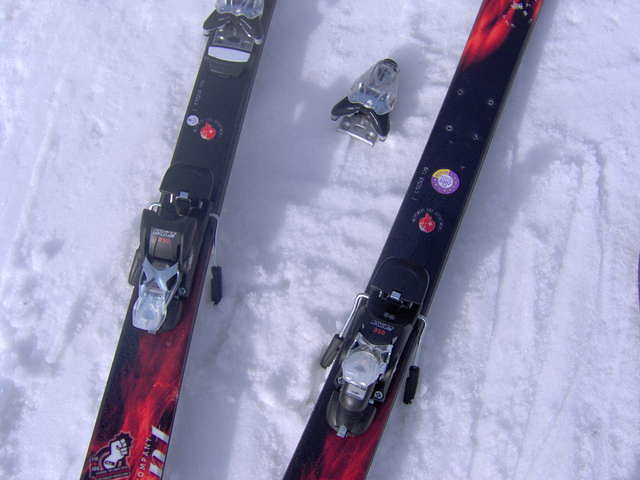In this close-up, overhead photograph, we see a pair of predominantly black and red downhill skis resting on well-packed snow. The ski tips and tails are out of frame, highlighting only the central portions where bindings attach. The snow is crisscrossed with ski tracks and footprints. The red patterns on the skis resemble flames set against a black background, punctuated with mostly unreadable writing and logos—one barely discernible word appears to be "company."

Attention immediately draws to the right ski, where the front binding is missing, revealing screw holes lacking their fasteners. The plastic guard and boot piece are also absent, suggesting a rough encounter possibly caused the binding to pop off. The disconnected toe piece lies between the skis. Despite the intact bindings on the left ski, there's no quick fix on the mountain, rendering the skier's day effectively over unless a ski shop is available nearby.